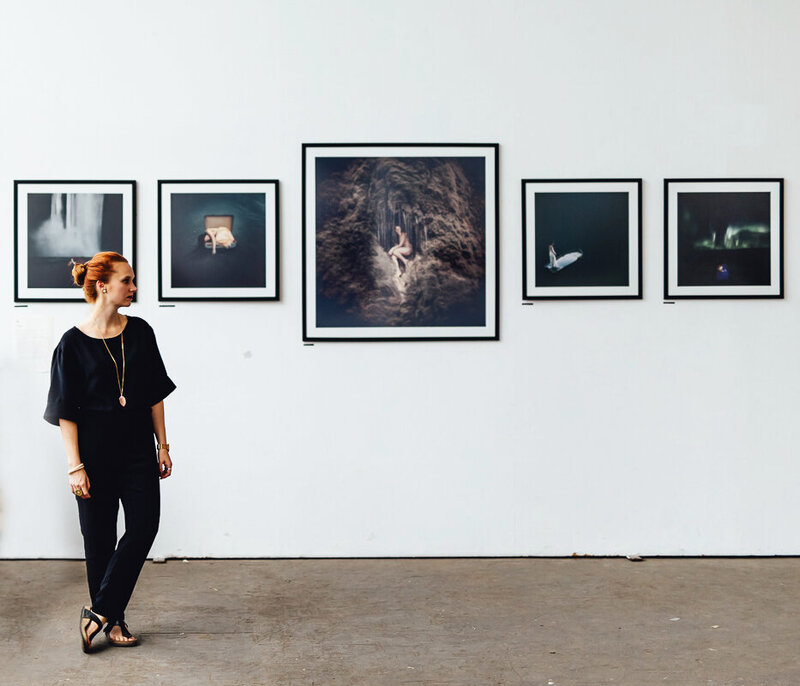The photograph captures a woman standing in an art gallery, positioned in front of a stark white wall adorned with five framed pieces of art. The floor beneath her is a brownish concrete. The arrangement of the artwork features a large square image in the center flanked by two smaller square images of the same size on each side. These pieces appear to depict various scenes involving water, a woman laying in water, and a woman at a waterfall, characterized by dark tones with hints of brown and blue. The central, larger image shows a woman, possibly nude, amidst mountains or rocks, while the surrounding smaller images continue a similar theme featuring the same woman in different serene and natural settings.

The woman viewing the art stands with a relaxed posture, one leg crossed over the other. She is dressed entirely in black, including a loose-fitting top that extends slightly past her elbows, black pants, and black sandals. Complementing her attire, she wears gold jewelry comprising a long necklace, earrings, bracelets, and rings. Her fair skin contrasts with her striking reddish-orange hair, which is styled into a bun. She gazes thoughtfully at the artwork, providing a poignant contrast to the minimalist, bright setting of the gallery.